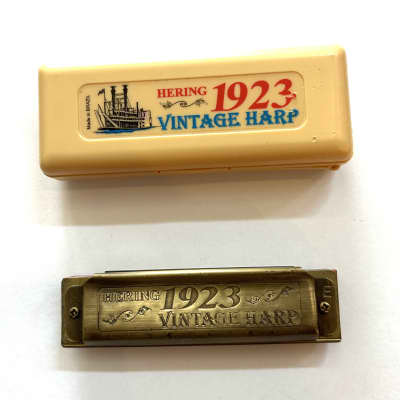This photograph captures a vintage harmonica and its carrying case, placed neatly on a plain white surface. The harmonica, labeled “Herring 1923 Vintage Harp,” appears to be crafted from a brass or copper-colored metal with an engraved logo that includes an illustration of a ship and the same text. The harmonica features a sophisticated design with two visible screws on either end, giving it a solid, aged appearance. Accompanying the harmonica is its vibrant carrying case, which is a pinkish-orange or yellowish plastic with the same “Herring 1923 Vintage Harp” branding. The case, complete with a ship logo, showcases red and blue text. The entire composition, lit from above, casts soft shadows on the white background, adding depth to the photograph. The focus of the image is the harmonica, which seems to bear the elegance and history of nearly a century, and the carrying case that protects it.